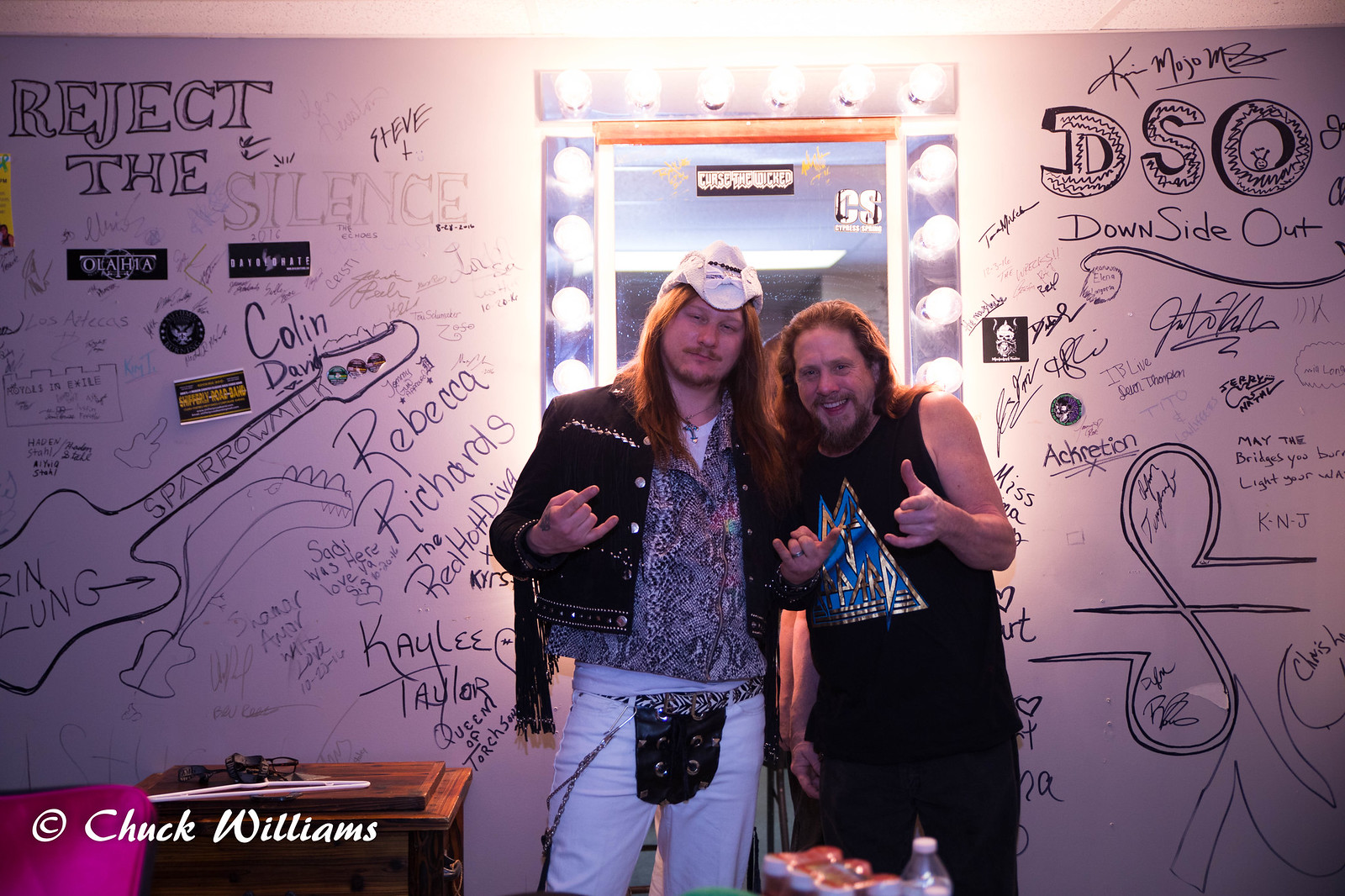In this horizontally aligned rectangular image, two men stand side by side against a cluttered wall covered in handwritten graffiti, signatures, and drawings made with black markers. The wall, suggesting a possible backstage or dressing room scenario, features a central mirror surrounded by bright white light bulbs for illumination. 

The man on the left wears light blue jeans, accessorized with a chain around his waist and a leather pocket attached to his front belt. He sports a white hat atop long, orange-ish brown hair, a tattooed right hand, and a black jacket adorned with fringe hanging from the sleeves. This man is throwing a peace sign with his right hand, embodying a rock and roll style.

To the right, his companion dons black pants paired with a black tank top featuring a blue and gold triangular design, suggesting it might say "Def Leppard." He also has long, orange-ish brown hair and thin facial hair, and is pointing forward at the camera.

The bustling wall behind them includes messages like "DSO Downside Out" in the upper right and "Reject the Silence" in the upper left, interspersed with names like Colin, Rebecca, and Richards, as well as an outline of a guitar. In the lower left-hand corner of the image, a white copyright symbol and the name "Chuck Williams" are visible.